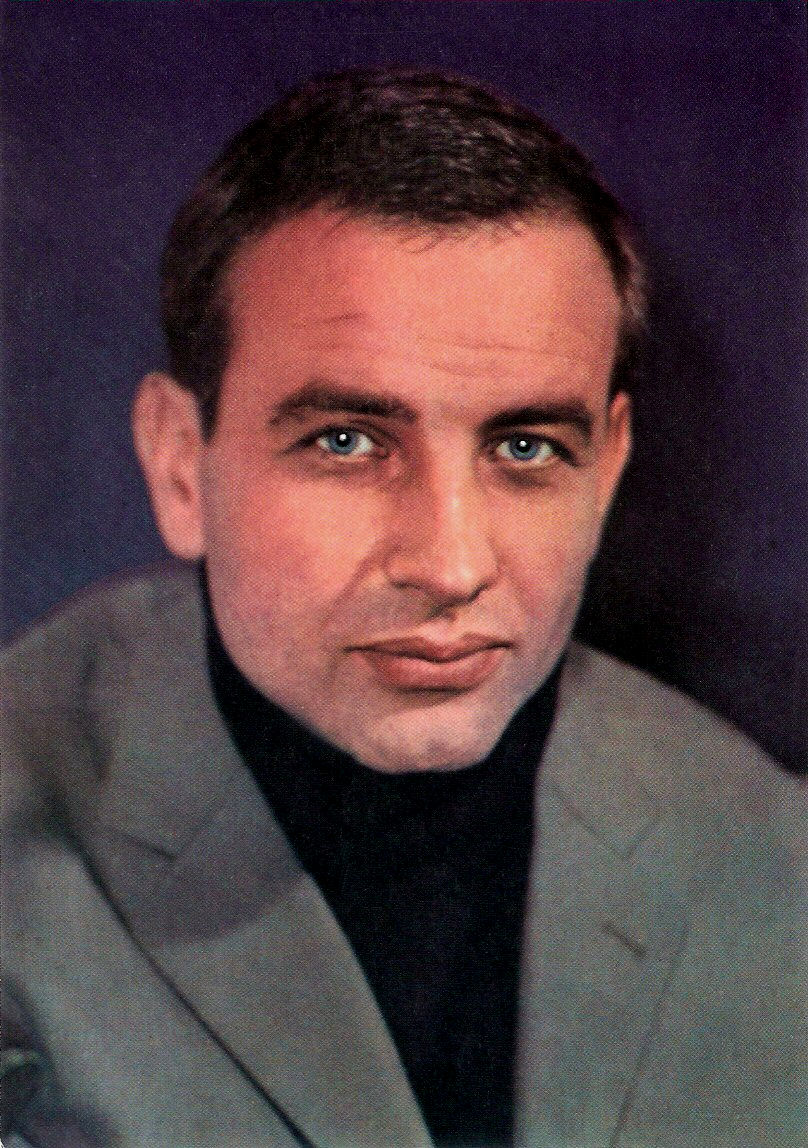The photograph displays a close-up of a man with short, dark brown hair and blue eyes, appearing to be of lighter skin complexion. He sports a serious expression and is slightly turned to his left, staring directly towards the camera. He is wearing a heavy grey wool suit jacket over a black shirt that extends up to his neck. His face is clean-shaven with just a hint of a 5 o'clock shadow. The backdrop behind him is dark blue with a slightly textured appearance, likely contributing to the image's grainy quality. Though the photo has a vintage look and is not perfectly sharp, it is clear enough to discern the man's features and attire. There are no other people, text, or numbers in the image, and it appears to have been captured using older camera technology.